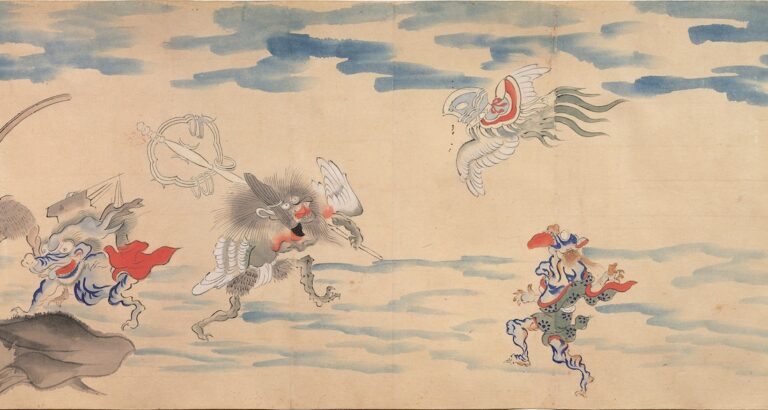The image appears to be a detailed, possibly old Japanese-style tapestry or painting on tan or beige canvas, showcasing a mythical scene. In the sky, there are blue clouds and four distinct figures, each with unique characteristics. One resembles a dragon, another a baboon, and a third is a flying creature with several tails. The fourth figure is a ghoul with a long tongue, depicted in blue. Below, there are additional figures, including one resembling a knight wearing a red cloak and another that appears to be a dragon. The background includes grey, blue, and red hues, with white wings visible on some figures, and a peculiar spoon-like object protrudes from one character's back. The tapestry has folds that are visible even in the minimized picture, adding to its antique and study-worthy appeal.